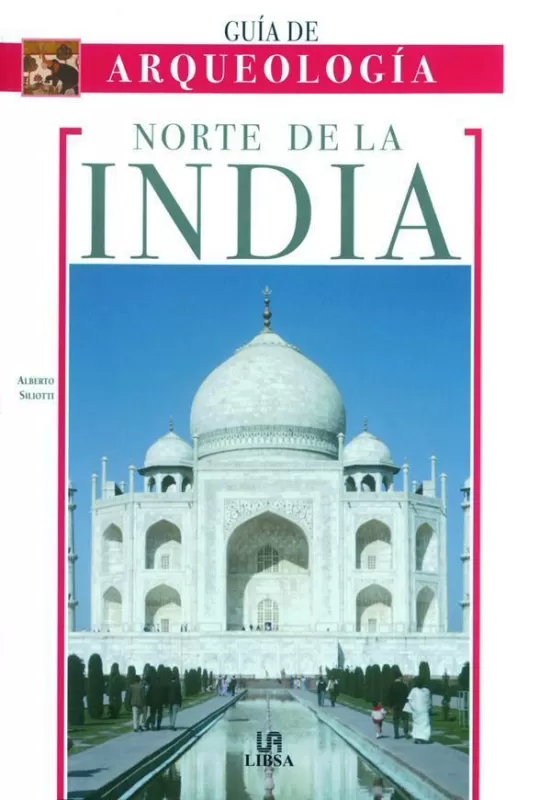The book cover prominently features a centered image of the Taj Mahal against a clear blue sky, its reflection mirrored in the pool of water stretching in front of it. On either side of the pool, there are people and tree-lined pathways. The cover is predominantly white, with a magenta color block at the top that reads "Archeologia" in white, all-caps font, accompanied by an ancient drawing or piece of artwork. Above the image of the Taj Mahal, the title "Norte de la India" is displayed in green all-caps font, with “Guia De” in smaller green all-caps font above it. To the left of the title, in small all-caps font, is the author's name, Alberto Siliori. Below the Taj Mahal image is the publisher's mark, "Limsa." The overall design uses a mix of magenta, green, and blue hues.